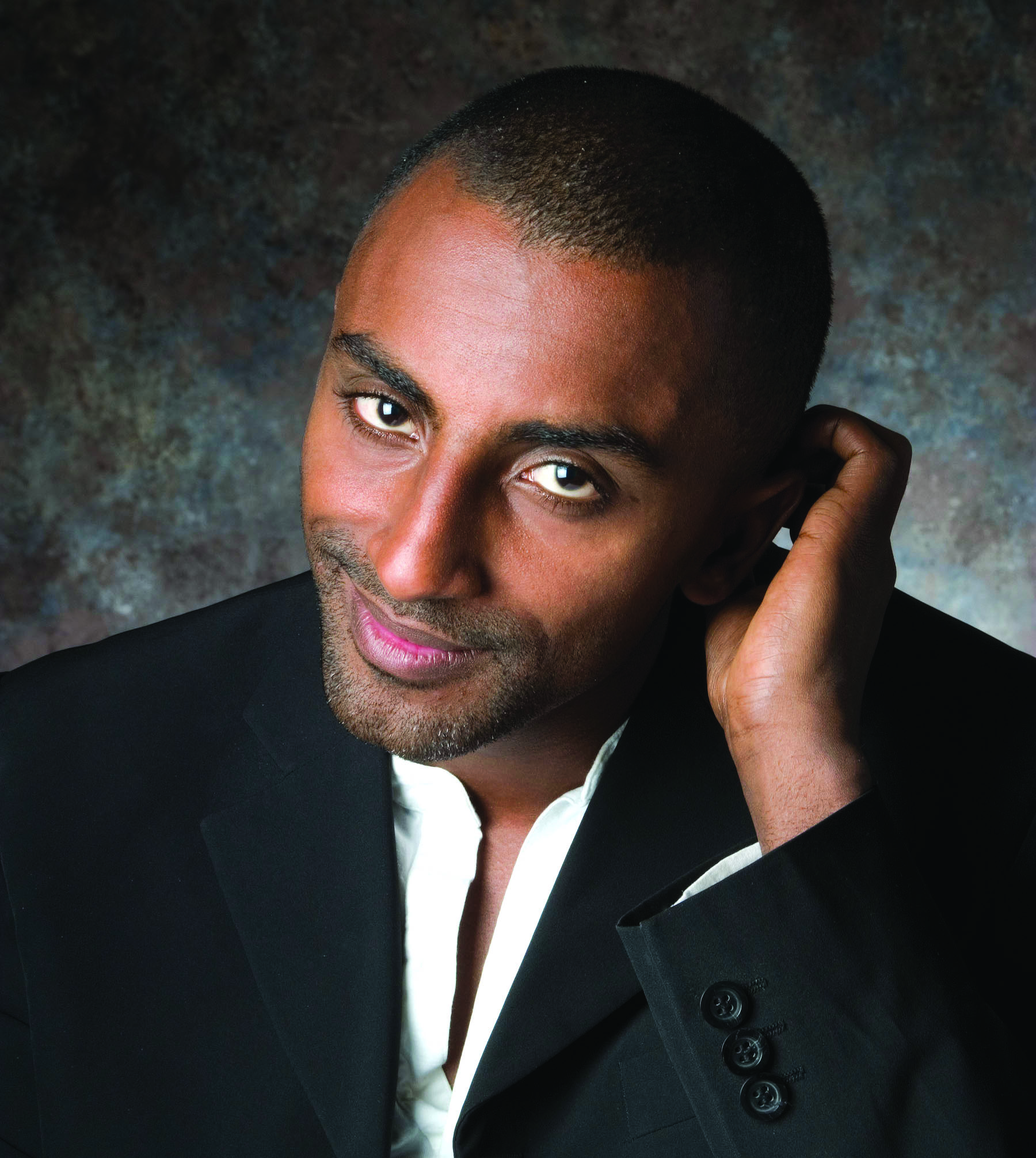The image depicts an African-American man posing against a marbled background featuring a blend of blue, gray, and reddish-brown hues. The backdrop appears to have splotches of paint, with areas darkening at the top and fading to lighter tones at the bottom, particularly brighter on the right side as if illuminated by a light source. The man is dressed in a black suit jacket with three visible black buttons on his right cuff, and he wears an open-collared white shirt beneath it. His short hair is buzzed, nearly shaved, and he has a bit of scruffy stubble forming a goatee with hints of gray. His eyes are dark brown, and he is smiling with closed lips. Notably, he raises his left hand up behind his ear, giving the impression that he might be scratching his head. His head is tilted slightly to the left, and he gazes forward and slightly upward with a dreamy expression.